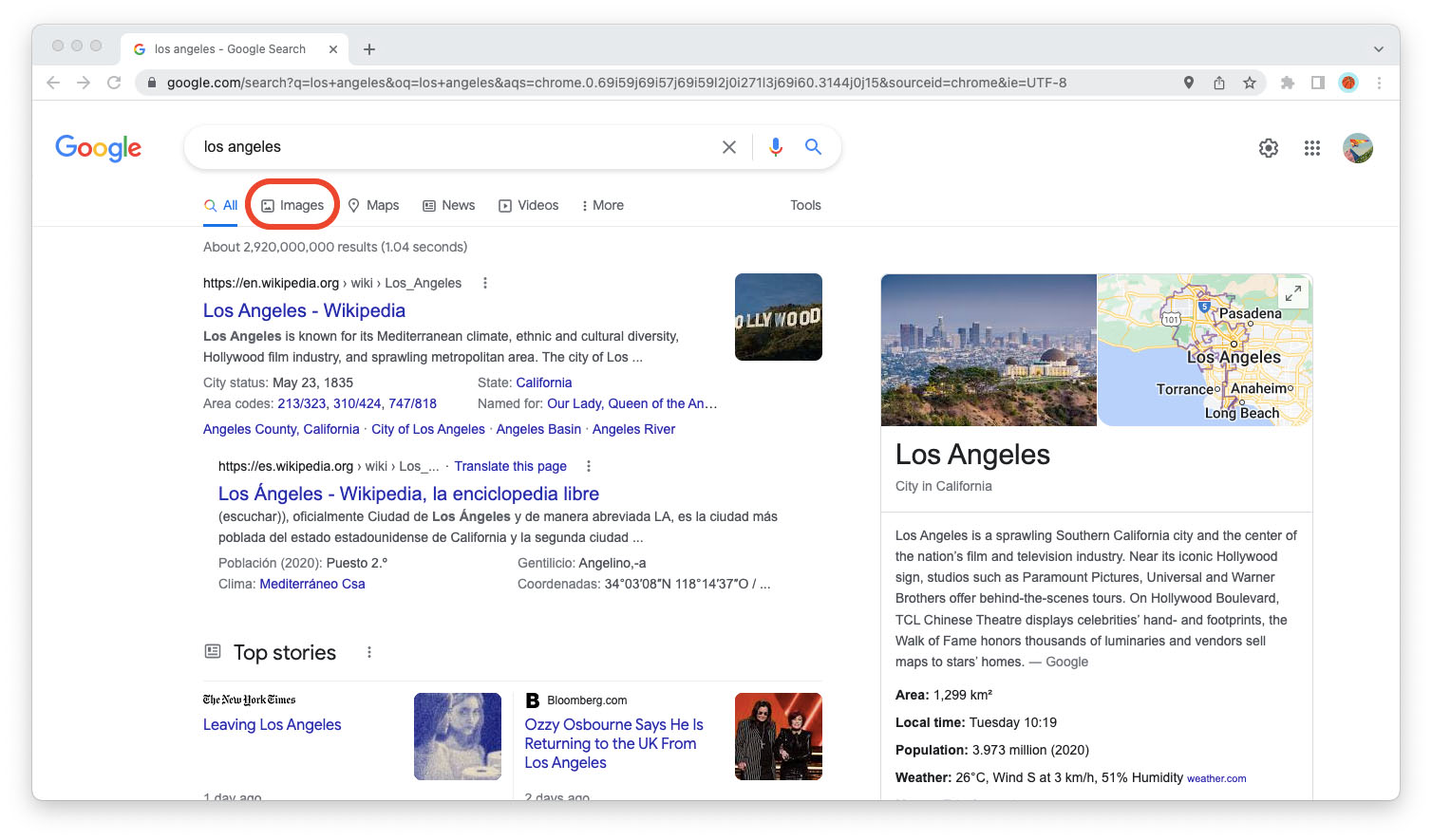This detailed screenshot captures the Google search page displayed on a MacBook. At the very top of the screen, the three standard control buttons for closing, minimizing, and maximizing the window can be seen, characteristic of a MacBook interface. Just below, a browser tab is labeled with the Google logo and the title "Los Angeles - Google Search." This tab has a close ('X') button and a plus ('+') symbol for opening a new tab. To the far right, there's a small downward-pointing arrow.

The next section showcases the browser's navigation bar, featuring a back button, a forward button, and a reload or refresh button. Adjacent to these is a lock symbol, indicating a secure connection, next to the URL bar. To the right of the URL, there are several icons: a location pin, a save icon, a star to bookmark the page, a puzzle piece symbol for extensions, a tablet icon, and a user profile symbol depicted in red. At the far end, three vertical dots provide access to additional settings.

Below this, the central portion of the screen features the Google logo prominently above a search bar containing the query "Los Angeles." There are options within the search bar to clear the text (via an 'X'), activate voice search (via a microphone icon), and initiate the search (via a magnifying glass icon). To the right, adjacent to the search bar, are a cogwheel for settings, a grid symbol likely linked to Google apps, and another red image, possibly linked to the user profile.

The webpage is segmented further down, displaying search navigation options. These include categories like "All," "Images," "Maps," "News," "Videos," and "More," with "Images" highlighted in red. The search results begin with a Wikipedia entry for Los Angeles, followed by another description possibly in Spanish. Below these entries, there is a "Top Stories" section with articles from the New York Times and Bloomberg.com featuring headlines about people leaving Los Angeles and Ozzy Osbourne returning to the UK from Los Angeles.

On the right side of the page, there's a visual section containing a picture of Los Angeles and a map of the city. Bold text reads "Los Angeles," followed by a subtitle “City in California” and a brief description or “About” section summarizing the city.